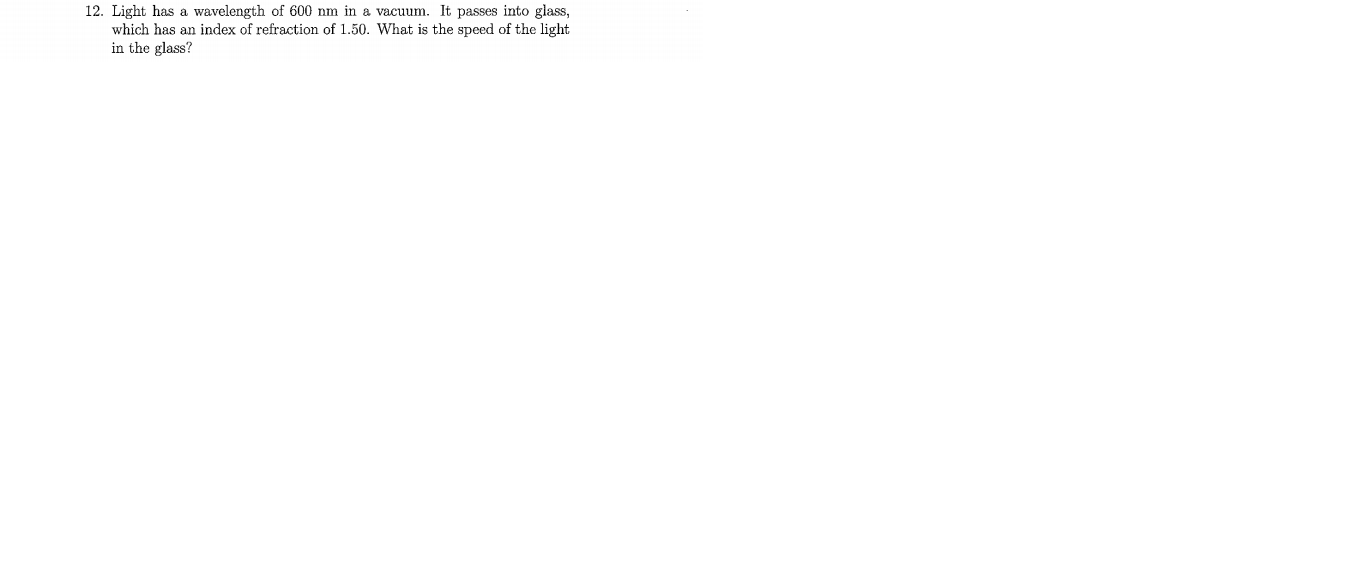The image predominantly features a blank white background, with a small, text-filled box in the center. Inside the box, there is a brief text that poses a question about the behavior of light. The text reads: "12. Light has a wavelength of 600 (the unit is not fully legible). In a vacuum, it passes into glass, which has an index of refraction of 1.50. What is the speed of the light in the glass?" The question is focused on calculating the speed of light as it transitions from a vacuum to a medium with a given refractive index.